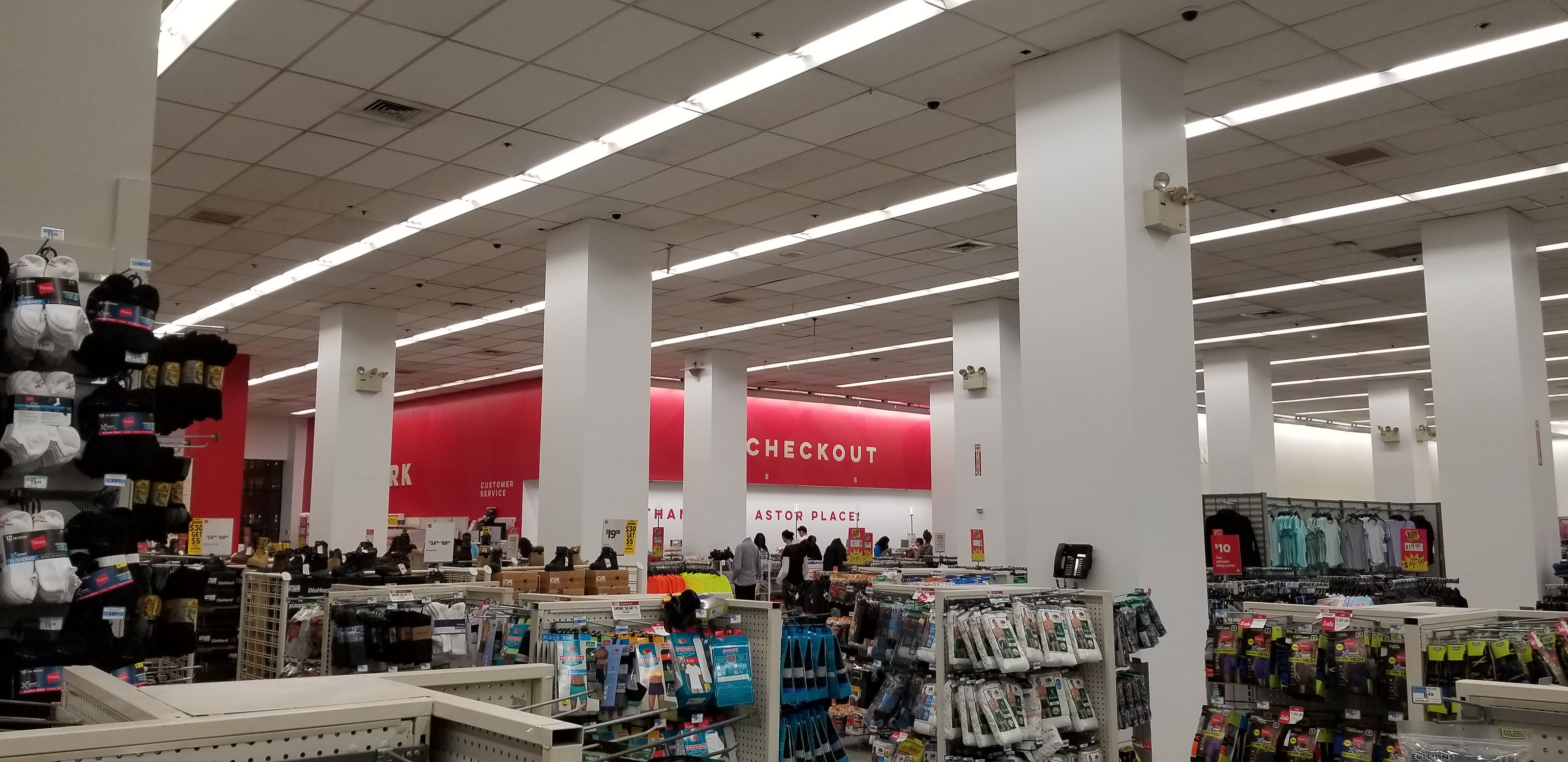The image depicts an interior view of a large retail store, possibly a Target, as suggested by the prominent red and white checkout signs—colors commonly associated with the Target brand. On the left side of the image, there is a wall densely packed with various types of socks. Adjacent to this, several displays feature men’s underwear, including packages of t-shirts and boxer shorts. Some displays may also contain gloves, although the image doesn't make this entirely clear. The store has large white columns positioned between the different displays, adding to the spacious, organized layout. Toward the back on the right side, a sign reading "Checkout" is visible, with a few people congregated in that area. The ceiling is constructed of square tiles, equipped with a few air conditioning vents for climate control. The overall atmosphere is typical of a large-scale big-box retailer, offering a wide variety of products in well-defined sections.